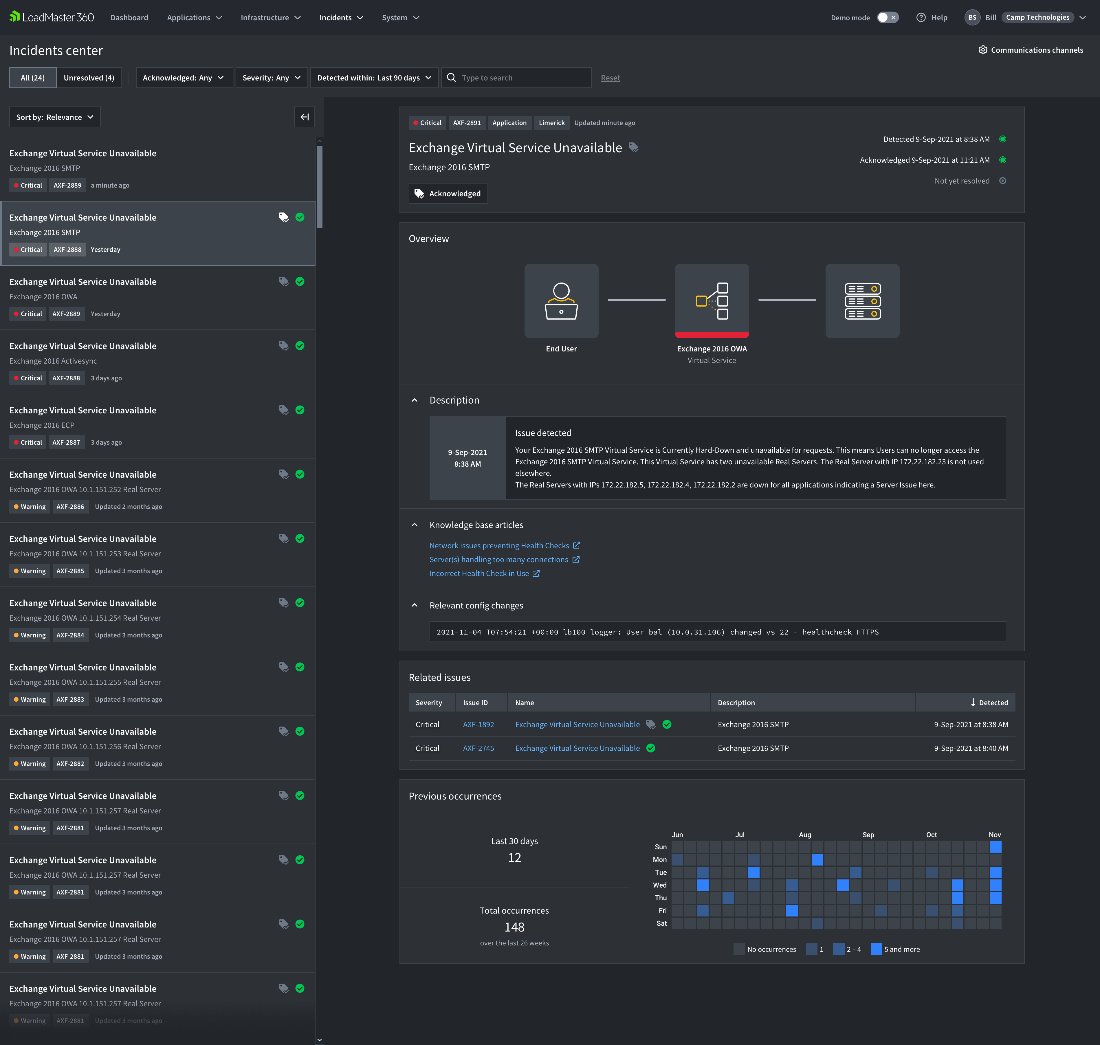The image depicts a computer screenshot in dark mode, showcasing a technical interface probably used for IT or network management. The screen features a predominantly black background with white and blue text. At the top center, it displays "CAD Master 360" and an "Incident Center" heading. Below this, a vertical column on the left side lists around 12 to 15 items, most of which repeatedly state "Exchange Virtual Service Unavailable." One of these menu items is highlighted, indicating user interaction with the menu labeled "All 34." 

On the right side, there are additional boxes also displaying "Exchange Virtual Service Unavailable." Below these, three distinct squares with icons are visible, each with its own label such as "Description" and "Issue," though the exact text is too small to read. Further down in the lower right corner, there is a chart composed of gray and blue squares.

This detailed screenshot appears to monitor various IT incidents, with the repeated "Exchange Virtual Service Unavailable" messages suggesting a widespread issue. The chart at the bottom likely visualizes data or the status of different services, adding further context to the ongoing incidents logged in this interface.